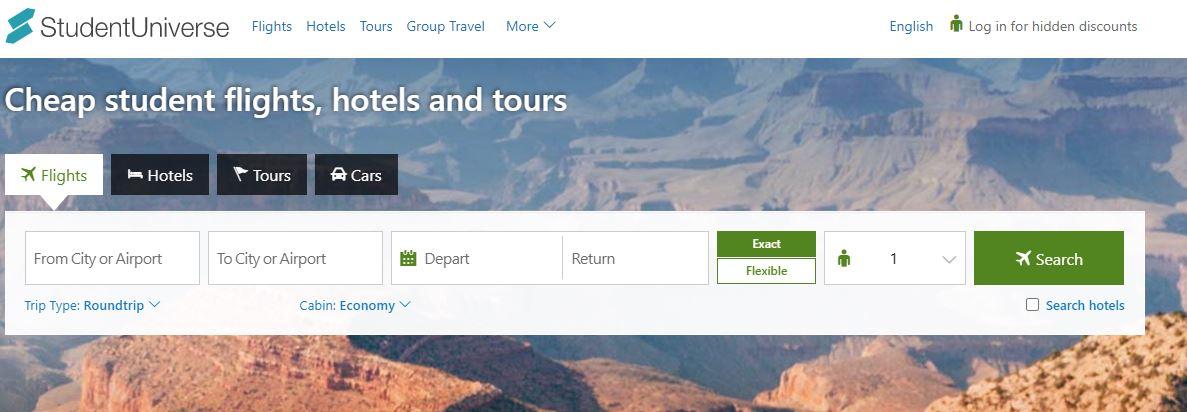A cropped screenshot of a web page displays a white banner at the top. On the top left, the text "Student Universe" is prominently featured, accompanied by a logo icon to its left. Adjacent to the name is text in blue that lists options: "Flights," "Hotels," "Tours," "Group Travel," and more. Further to the right, the word "English" appears, followed by a small person icon and the phrase "Log in for hidden discounts" in gray text located at the far right corner.

Below this banner, the body of the web page shows a scenic photograph of the Grand Canyon, which serves as a background for the web page information. Overlaid on this image, in the top left, is the white text, "Cheap Student Flights, Hotels and Tours." Below this header, there are four interactive boxes aligned horizontally. The first box, labeled "Flights," is highlighted in white, indicating it is currently active. Beneath the "Flights" box, a form is displayed, which includes fields for "From City to Airport," "To City to Airport," "Departure Date," and "Return Date." It also offers options for "Exact" or "Flexible" dates, a dropdown box to select the number of travelers, and a prominent "Search" button.